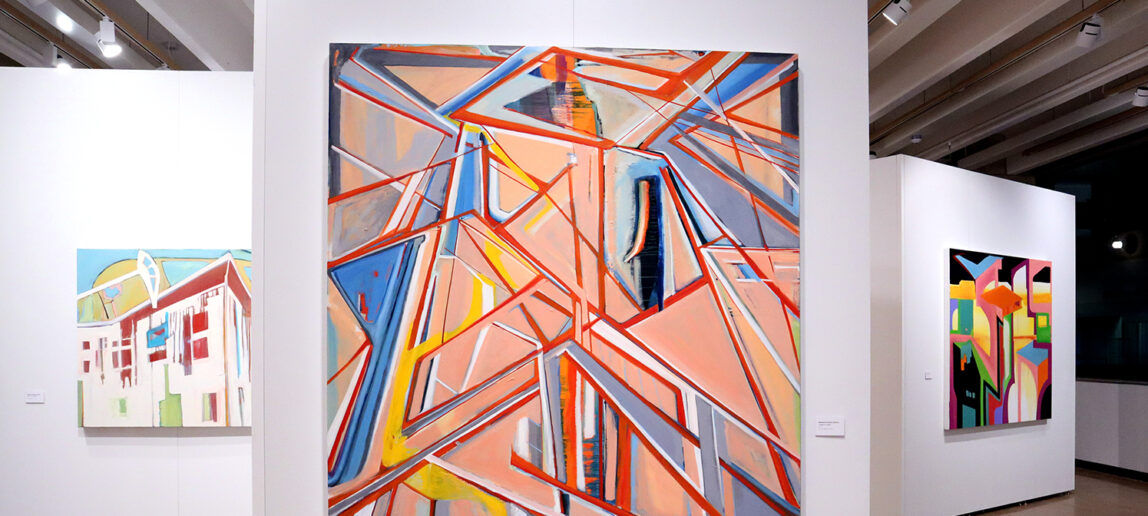In the photograph, an art museum or gallery is featured, showcasing a collection of modern and abstract artworks. Dominating the foreground is a large, central painting nearly the size of the white wall it is displayed on. This vibrant abstract piece captivates with intersecting orange lines creating a dynamic tapestry of triangles and rectangles, filled with a variety of colors including blues, yellows, and peach tones. The composition evokes an urban, graffiti-like aesthetic. To the left, a smaller painting portrays a stylized building, characterized by a white structure with cherry red accents and a sky segmented into yellow and light blue portions. On the right, another abstract painting mirrors the central piece’s style with geometric shapes and a vibrant palette incorporating pink, green, yellow, black, and light blue. The ceiling above features spotlights designed to enhance the artworks, confirming the setting as a professional art exhibit.